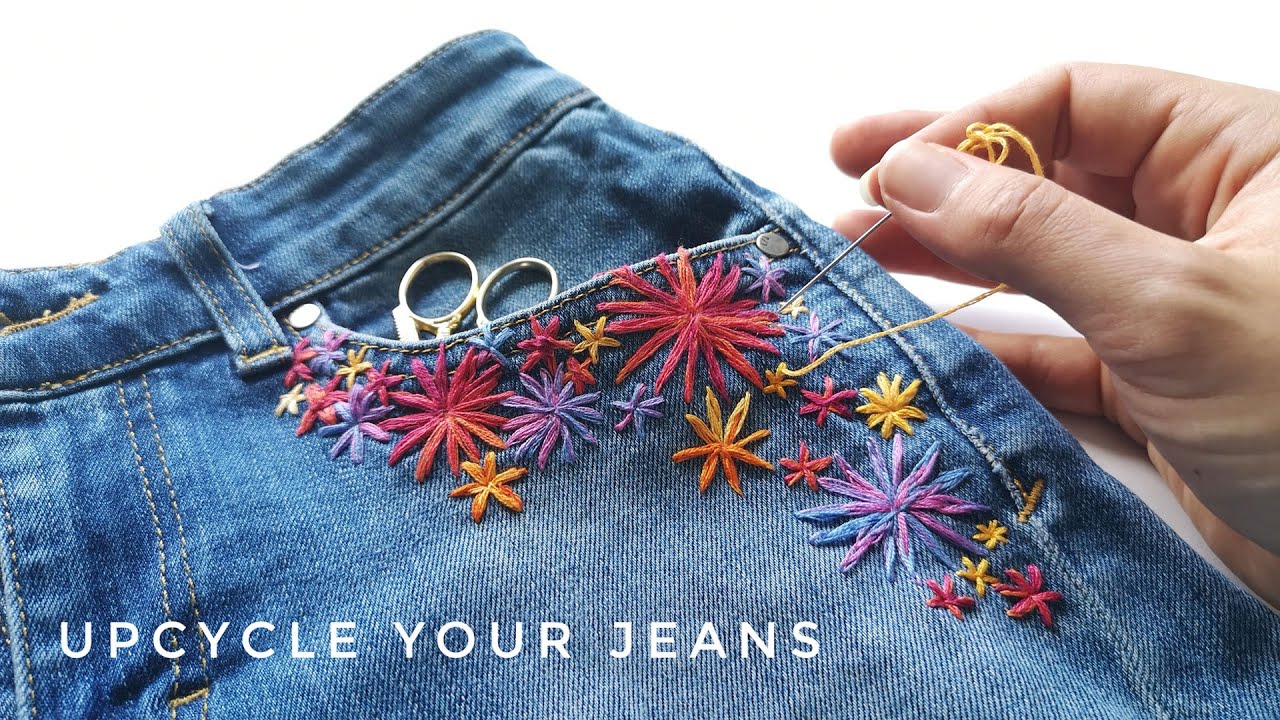The indoor photograph captures a rectangular image of a pair of blue jeans against a plain white background, blending into the screen without a border. The focus is on the left pocket of the jeans, where a gold-colored pair of scissors partially protrudes. A close-up of a Caucasian female hand is visible on the right side of the image; her pinky rests on a white table as she carefully sews multi-colored flower and star patterns onto the fabric with a needle and thick yellow thread. The small detailed stars and flowers are displayed in vibrant hues of purple, pink, yellow, and blue, embellishing the jeans artistically. Text in large white capital letters at the bottom left corner reads "UPCYCLE YOUR JEANS."